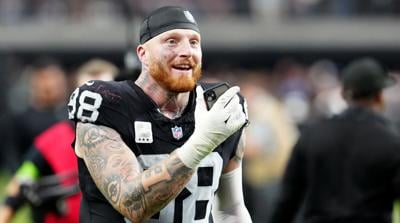This horizontally aligned, rectangular photo captures a professional American football player with a medium-length ginger beard and tattooed right arm, smiling broadly in the midst of a busy, blurred background, which appears to be a football field during daytime. Wearing a black jersey with the number 88 in large white text on the chest and sleeves, he is likely a Raiders player. He holds a cell phone in his white-gloved right hand, possibly FaceTiming or calling someone, and wears a tight black cap. The background features indistinct figures and structures, with a man in black on the right and a man in red and green on the left, emphasizing the lively atmosphere.